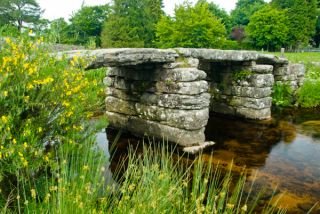The image depicts an ancient-looking stone bridge, predominantly gray and appearing somewhat weathered with patches of green, possibly due to algae or other vegetation. This human-made bridge spans a small river or creek, the water of which appears brown and yellow, perhaps from sediment. 

On the left side of the image, tall grasses and bushes with long fronds and yellow flowers grow densely, almost taking up half of the frame. The tall grass also surrounds the bridge area, suggesting a marshy environment. In the background, lush green trees stretch into the distance under a white sky, enhancing the natural outdoor setting of the scene.